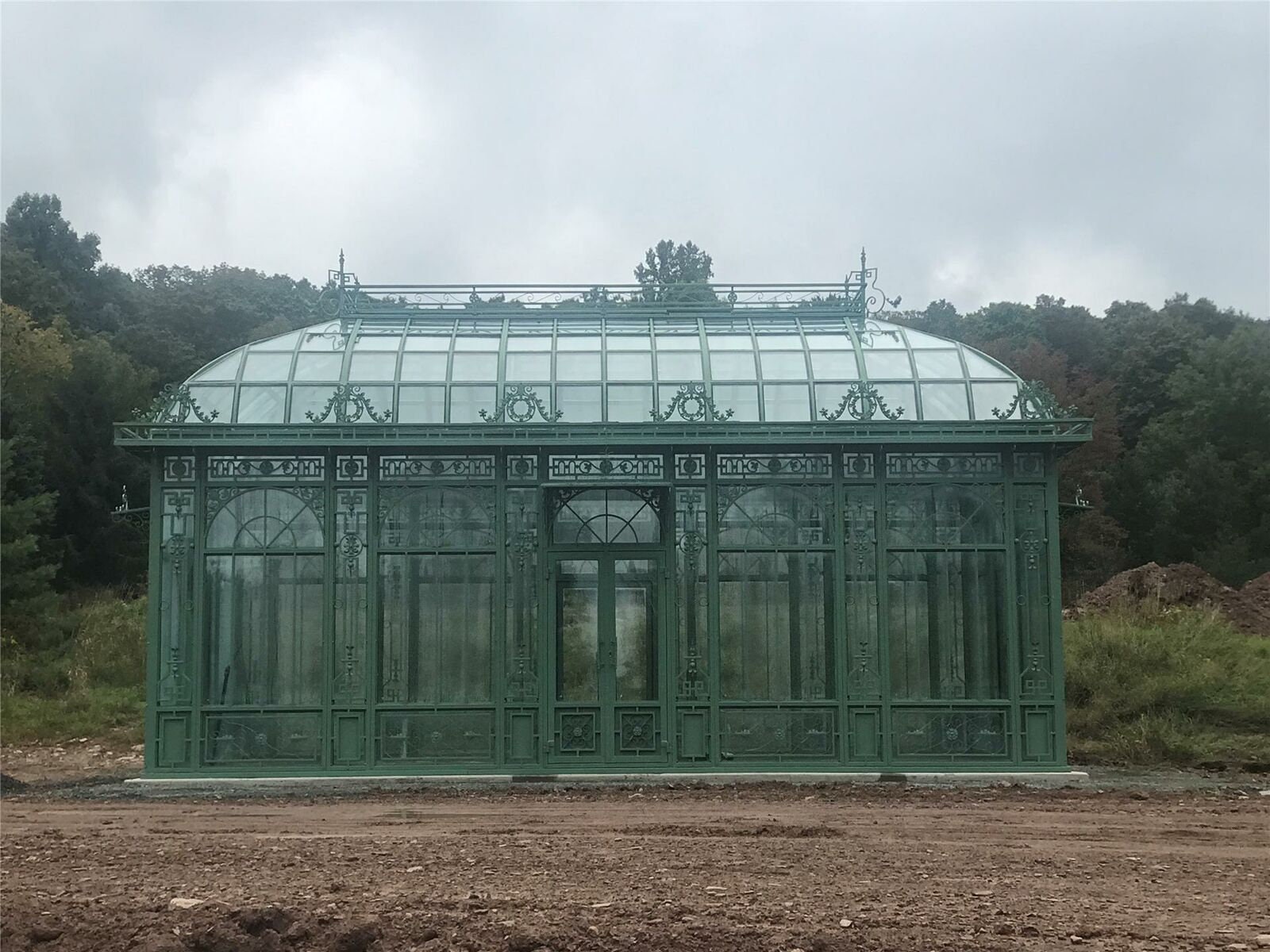This photograph captures a tall, vintage-style greenhouse, centrally positioned in the image. The structure is primarily composed of green metal and features a glass roof and numerous glass windows, allowing for ample transparency. The building sits on a concrete slab amid a dirt road or gravel area strewn with rocks. Despite its ornate doors and historical construction, the greenhouse appears to be empty. 

Behind the greenhouse, a dense row of large, verdant trees stretches from left to right, with some branches extending over the structure. Surrounding the area is undeveloped land with patches of green grass. Above the scene, the sky is overcast, filled with white clouds against a backdrop of light blue. This picturesque setting is devoid of any text or labels, focusing solely on the timeless architecture of the greenhouse and its natural surroundings.